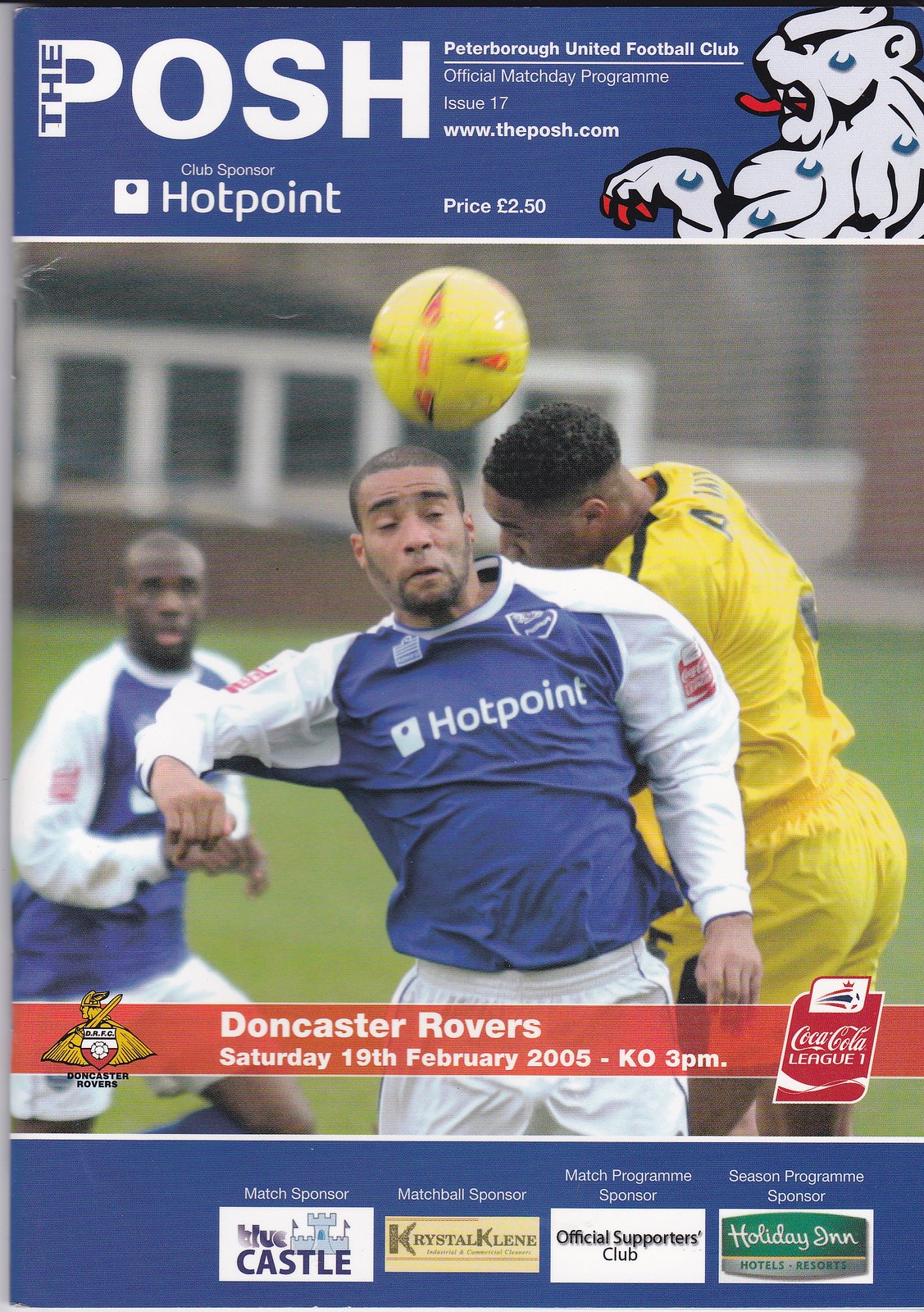The image is the cover of a sports program for a soccer match between Peterborough United and Doncaster Rovers held on Saturday, 19th February 2005. At the top of the cover, a blue banner displays the word "POSH" in white, with the letters "THA" in blue incorporated into the "P". To the right, it reads "Peterborough United Football Club Official Match Day Program Issue 17" alongside the club's website, www.theposh.com, and the price, £2.50. There is also a white mountain lion icon on the right-hand side, associated with the club sponsor Hotpoint.

The main photo on the cover is set against a mixed green and brown background and shows three soccer players in action. In the foreground, a man in a blue jersey with white sleeves and white shorts is seen with a tense expression, eyes closed, and mouth cringing, attempting to head a yellow ball just above his head. Directly behind him, another player in the same blue kit looks on, slightly crouched. Further back, a player in an all-yellow kit is seen sideways, also appearing to track the ball. In the blurred background, there are windows and what appears to be grass. At the bottom of the cover, another blue band is present with "Doncaster Rover" written across a red bar underneath.